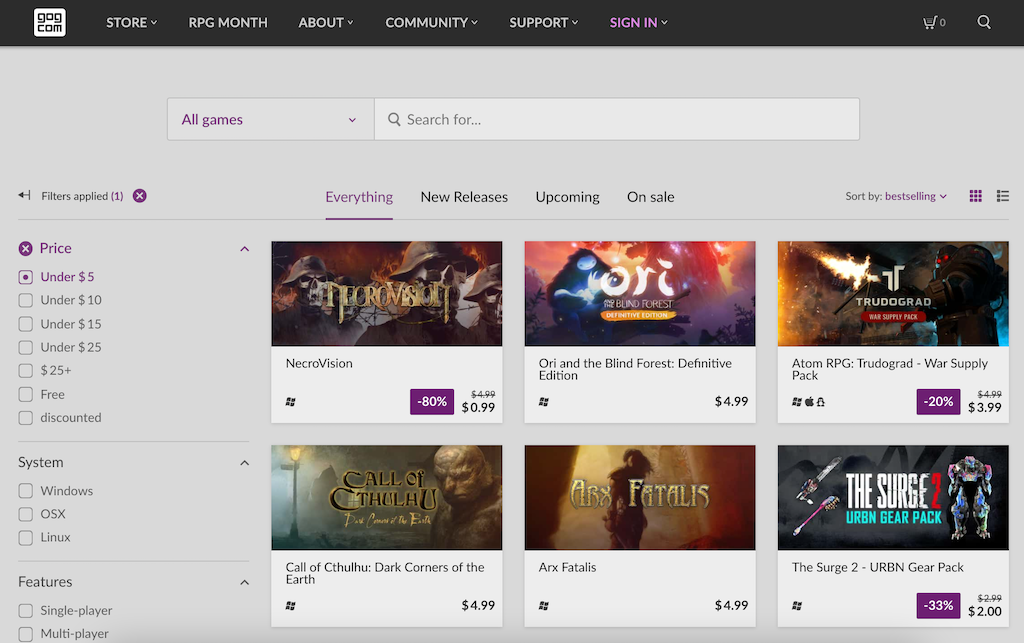The image captures a screenshot from a webpage, specifically from the back end or a section of it. At the very top of the page, there is a banner with the website name "GOG.com" prominently displayed. Adjacent to this, in a white rectangular box, are various navigation options labeled: Store, RPG Month, About, Community, and Support. Additionally, there are icons for signing in, a shopping cart, and a magnifying glass symbolizing search functionality.

Below the main banner, an organized menu provides more options including All Games, a search bar labeled "Search for...", and multiple tabs signifying different categories. The currently selected tab, highlighted in purple and underlined, reads "Everything," indicating comprehensive browsing. Alongside it are tabs for New Releases, Upcoming, and On Sale.

Moving further down, the page features a grid displaying six video game titles available for purchase. The first row includes "NecroVision," "Ori and the Blind Forest: Definitive Edition," and "ATOM RPG: Trudograd." The bottom section of this grid lists additional titles, although it specifies that there are three more games in this row without providing their names.

The layout suggests a structured and user-friendly design, aimed at facilitating easy navigation and discovery of games for potential buyers.